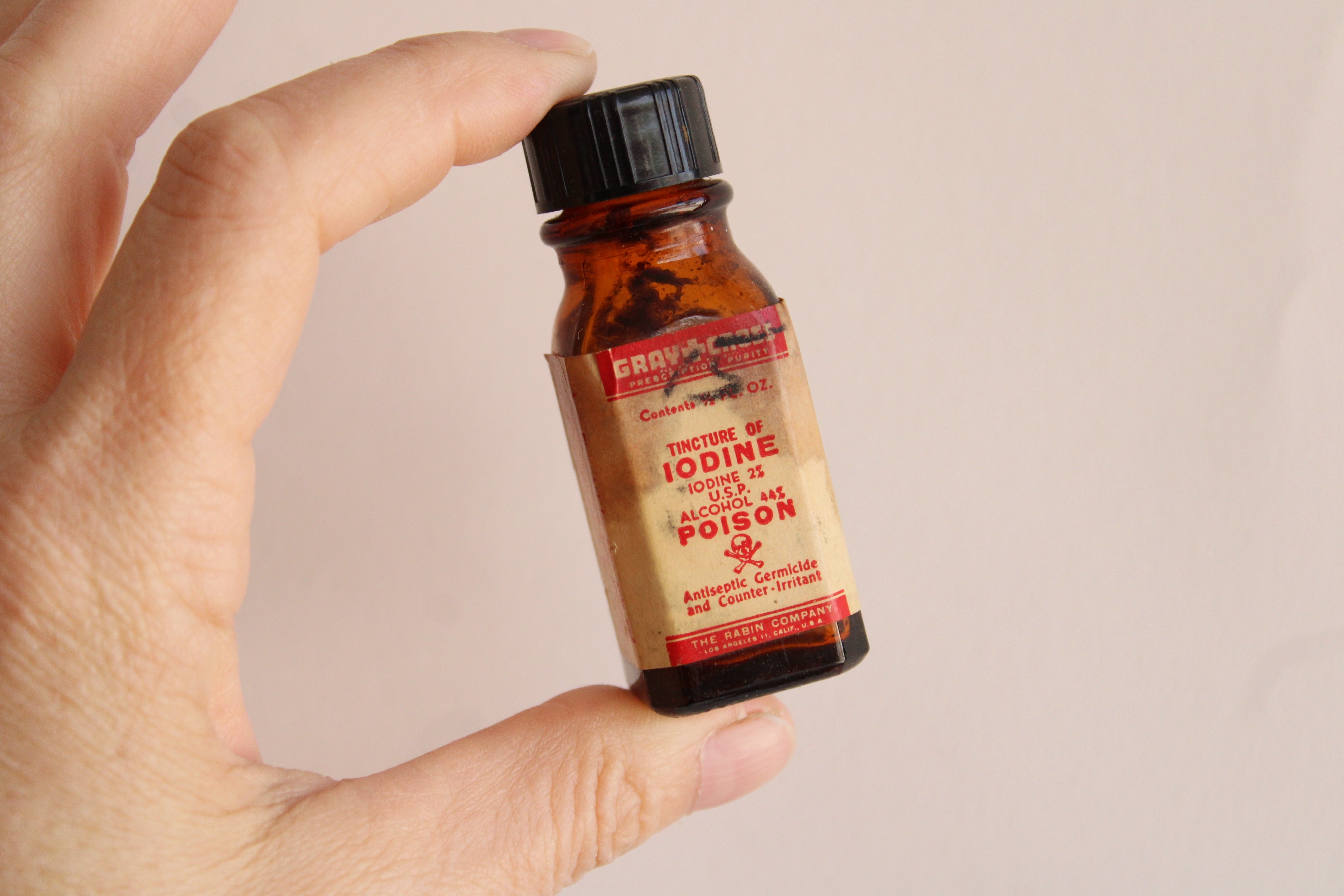In a horizontally rectangular, full-color photograph with an artificial light source and a very light purple, almost beige background, a partially visible Caucasian hand is holding an old glass bottle of iodine. The hand appears on the left portion of the image, with the thumb, index, and middle fingers grasping the bottle gingerly in a C shape. The bottle itself is brown with a black lid, and it has a very worn, cream-colored label with red print. This label features various inscriptions, including "tincture of iodine," "2% USP alcohol," "44% poison," "antiseptic, germicide, and counterirritant." There are crossed-out details with the handwritten number "15" over some text. A red skull and crossbones symbol indicating poison is prominently displayed, along with the name "The Rabin Company, Los Angeles, California, USA" at the bottom. The label shows signs of aging with noticeable stains.